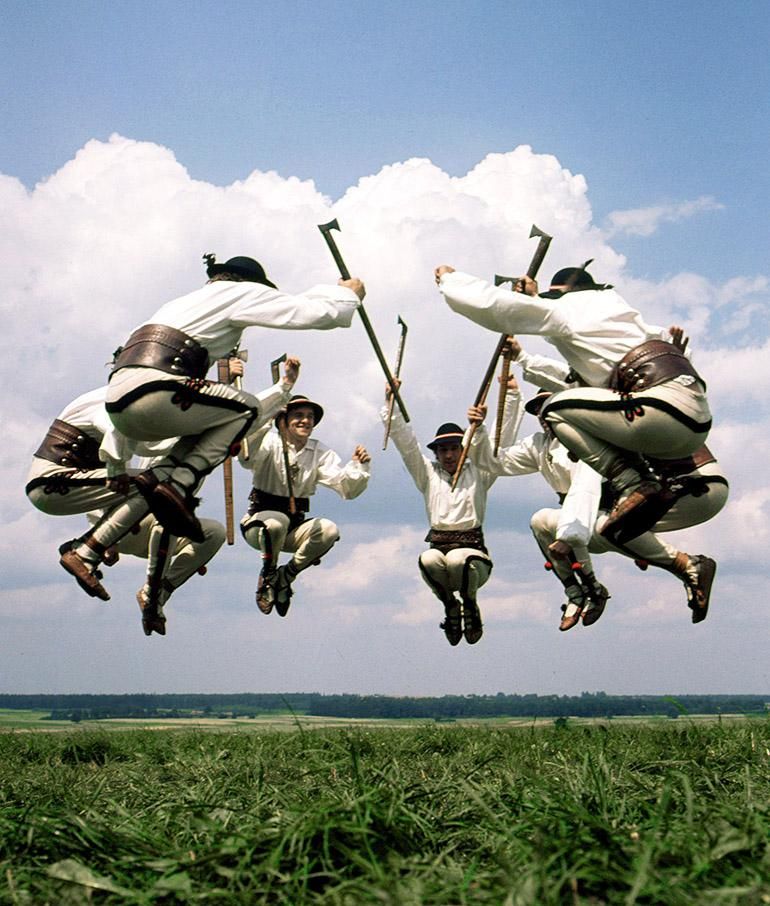This photograph captures a group of eight men, mid-jump, in a tightly synchronized formation over a closely-cut grassy field that stretches to the horizon. They are dressed in traditional German highland attire, featuring white frilly shirts, white breeches, brown leather belts, and brown shoes. Each man wears a distinctive hat adorned with a feather, and small red pom-poms decorate their knees. They all hold small hatchets in their right hands, the blades glinting in the daylight. The backdrop consists of vivid green grass, which transitions into a strip of yellow and then a distant line of green trees. Above, the sky is a brilliant blue, adorned with fluffy white clouds. This image, devoid of any text, beautifully captures the essence of their cultural ensemble and spirited leap.